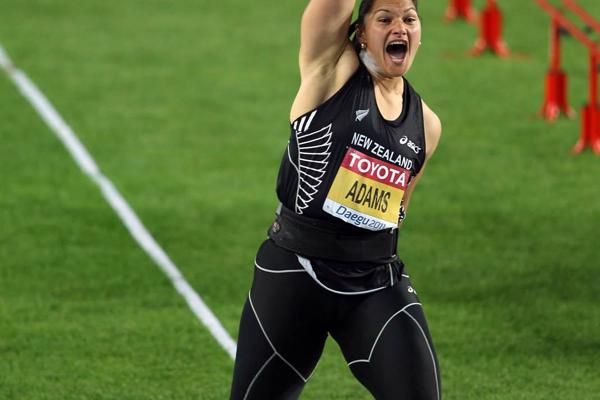In this photograph, a female athlete named Adams is celebrating triumphantly on a green grass athletic field. She is wearing a black tank top adorned with sponsors, prominently displaying "New Zealand," "Toyota," and her name, "Adams," on a yellow box. Her outfit includes blue athletic tights and possibly black shorts. She exudes elation with her mouth wide open in a victorious yell, and her right arm raised high in the air. The background reveals a white line on the field, emphasizing the sports setting, along with red guardrails or hurdles visible in the top right corner. The image captures the intense emotion of her success in the event.